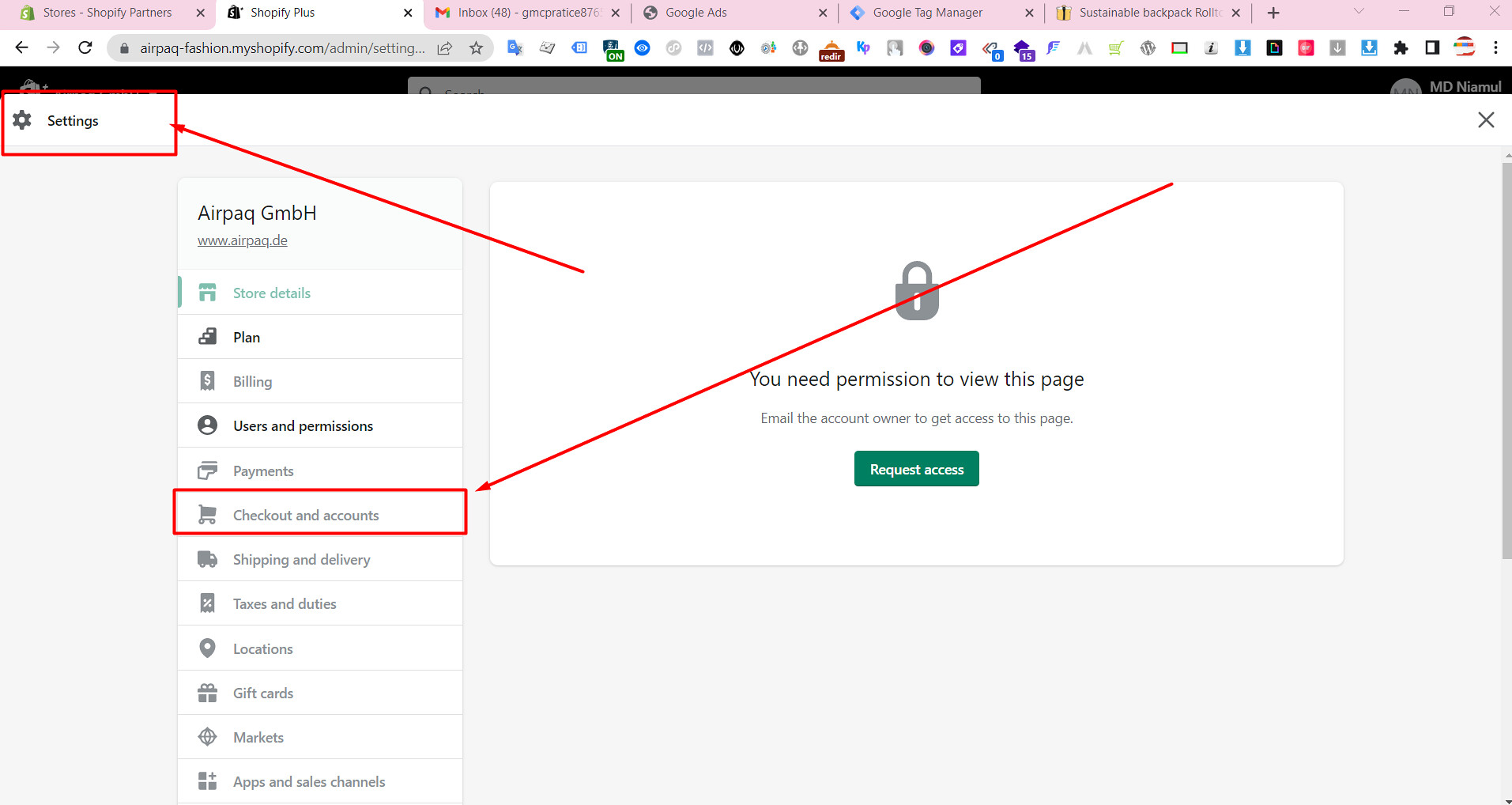A screen capture showcases the settings page of the Shopify Plus app on a computer screen. In the upper-left corner of the image, the settings icon is prominently highlighted with a red rectangle and an accompanying red arrow, drawing attention to its location. Among the various menu options visible in the settings, the "Checkout and accounts" section is also distinguished with a red rectangle and arrow, indicating its significance. Centrally located on the screen is a security message featuring a padlock icon. Below the icon, the message reads: "You need permission to view this page. Email the account owner to get access to this page. Request access." This captures the importance of requiring proper authorizations to proceed.